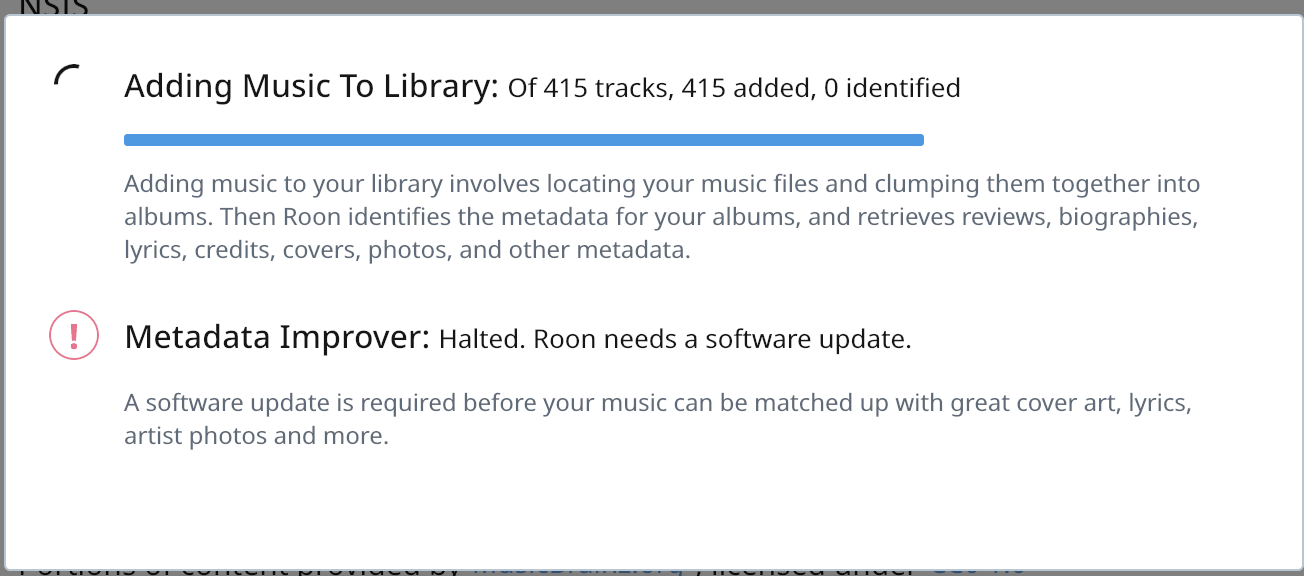The image depicts a user interface screen with a white background and a solid blue line running horizontally beneath the text "Adding music to library of 415 tracks." It indicates that 415 tracks have been added, with zero identified. The primary text is written in black. There is also a red exclamation point circled, with the red text "Metadata improvement halted. Room needs software update." This additional information is listed in grey. Surrounding this interface is a grey border, with a thin blue line on one side. Black initials, too illegible to read, are present at the top of the screen.